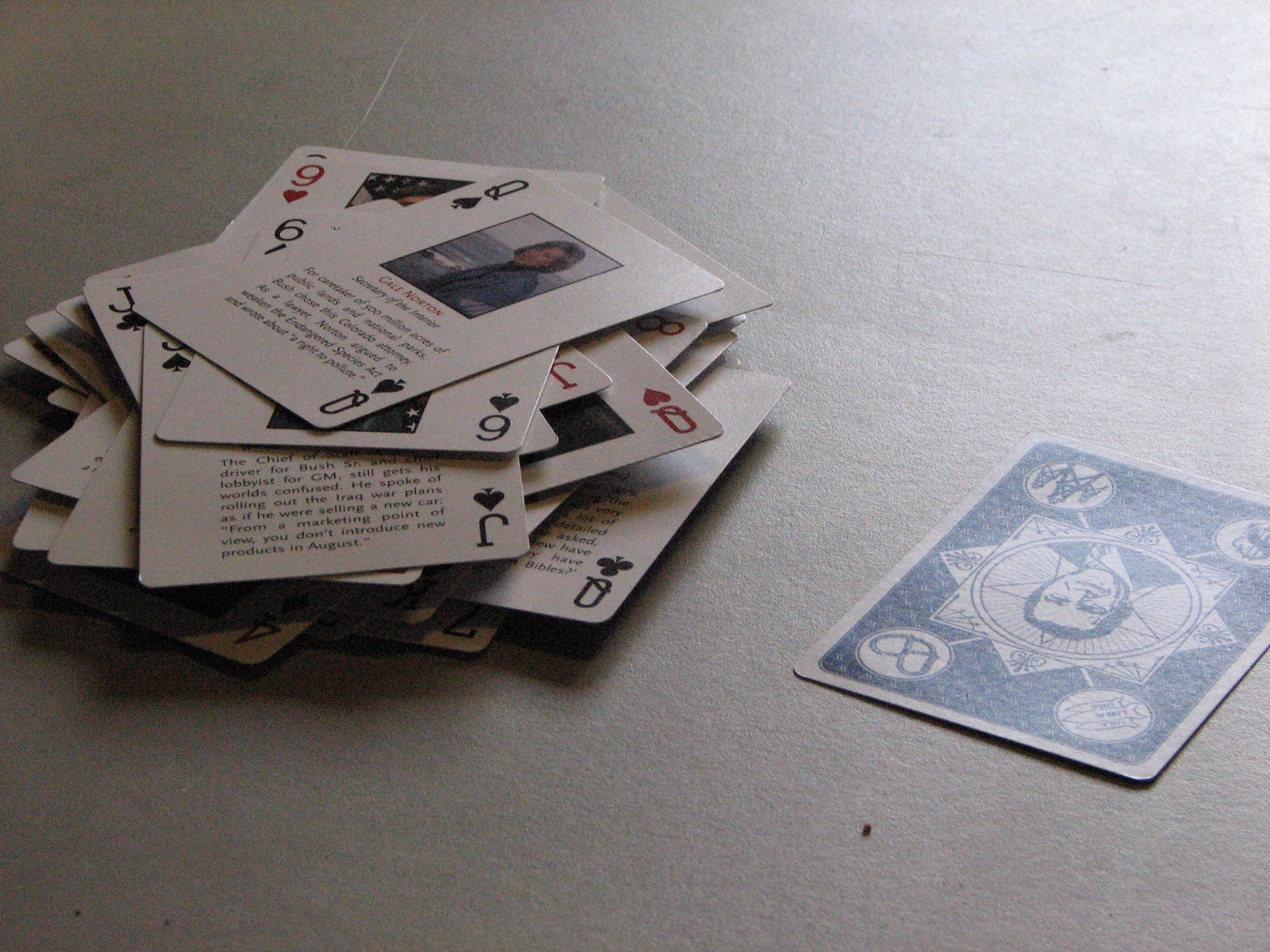This close-up photograph captures an intriguing collection of playing cards on a whitish surface. At a slight angle and upside down, a single card takes center stage. Unlike standard American decks, this card features a grainy black and white design. The central image showcases a distinguished gentleman from the chest up, clad in a suit and tie.

To the left of this card lies an untidy stack of similarly unique cards, haphazardly fanned out in various directions. At the top of the disordered pile is the Queen of Spades, a card predominantly white with striking black details. The upper section of this queen card reveals an image of an elegant woman with a bluish-gray ocean landscape behind her. Below this image, red and black small print adorns the card, culminating in a concise black-printed paragraph at the bottom.

This detailed arrangement suggests that the entire deck features individual cards, each with varying images, text, and numeric values, creating a visually rich and complex tableau.